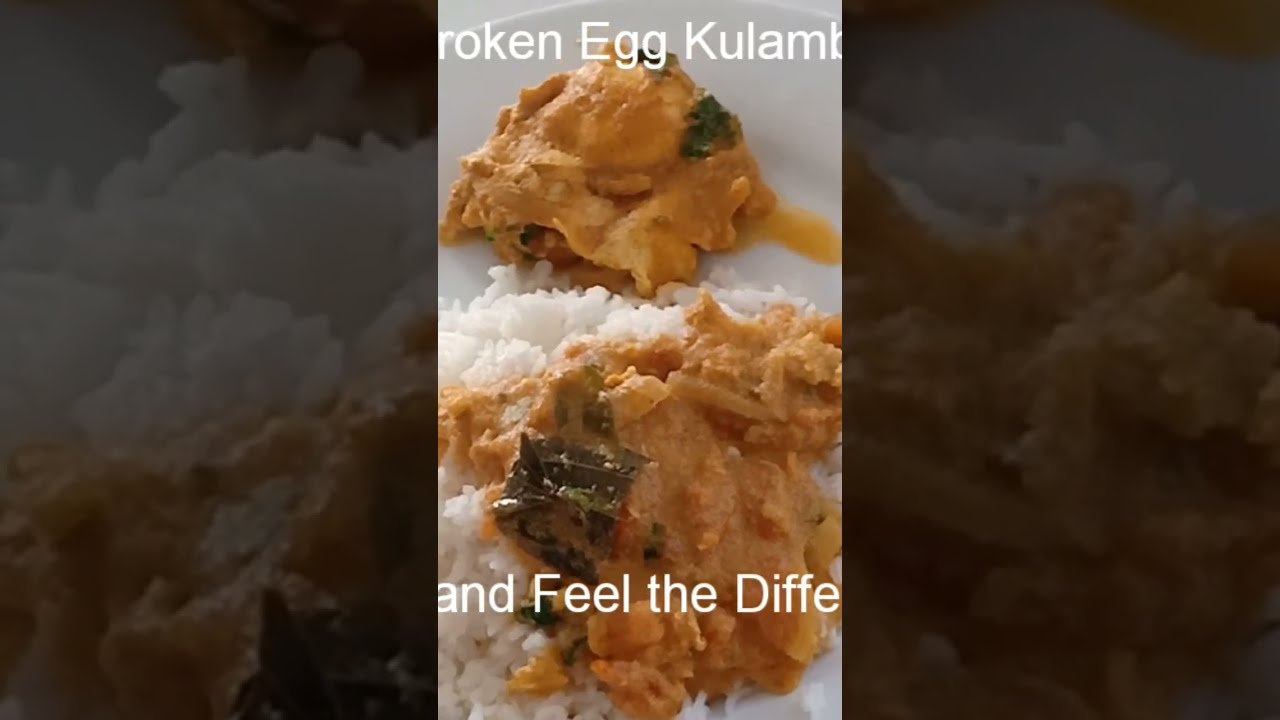The image features a close-up screenshot of a dish on a large circular white plate, likely taken from a mobile app such as TikTok or Instagram Live. The dish consists of a mound of white rice topped with a beige, orangish-brown curry, which includes chunks of meat, possibly lamb, and green leafy vegetables, likely grape leaves. There are also some visible peanuts scattered within the curry. The plate occupies almost the entire frame of the rectangular photo, which is formatted to the size of a phone screen. Text overlays the top and bottom of the image: the top reads "Broken Egg Kulamb" and the bottom states "and feel the difference," suggesting it is an advertisement, possibly for a cooking channel.